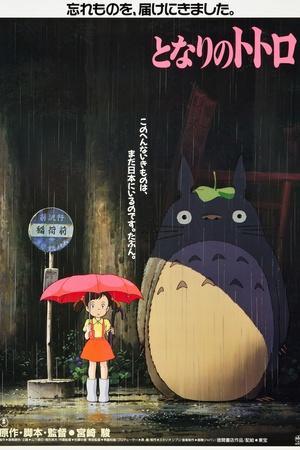This image is a highly detailed illustration, likely serving as a cover for a comic book or a poster for the beloved anime movie "My Neighbor Totoro." The text on the image is in an unfamiliar language, potentially Korean or Japanese, and is typeset in pink in the top right corner using unique symbols. The scene depicts a rainy day where a small girl, dressed in an orange jumper over a yellow top, stands in white rain boots while holding a red umbrella. She is positioned next to a blue, round sign, suggestive of a bus stop. To her right stands Totoro, the iconic large creature with a large belly, pointy ears, and white eyes with black pupils. Totoro is partly in shadow and has a distinctive leaf atop his head, serving as an inadequate umbrella. The background hints at a bench, reinforcing the bus stop setting, adding to the image's charm and depth.